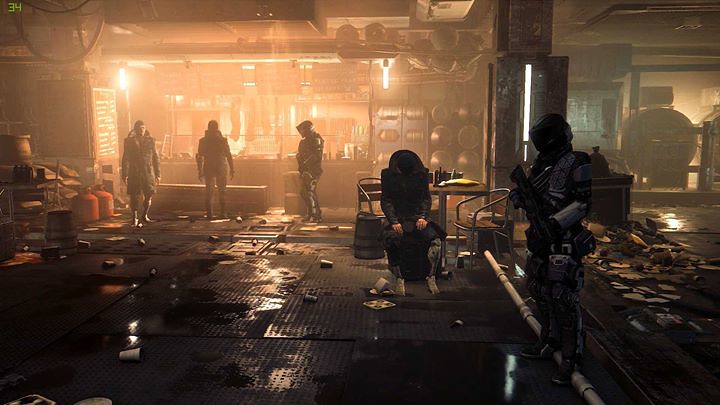This screenshot appears to be from an action video game, depicting the dimly lit interior of a building that resembles a trail or corridor. On the right-hand side, a character is visible holding an automatic weapon pointed slightly downward, presenting no immediate threat. In the center, another figure sits on a chair with his head bowed, dressed in black attire, with light-colored feet and hands resting in his lap. The background suggests the setting might be a bar, illuminated and featuring three other characters adorned in Western military garb. The floor of the area is cluttered with debris, watermarks, and scattered cups and spilled liquids, adding to the chaotic ambiance.